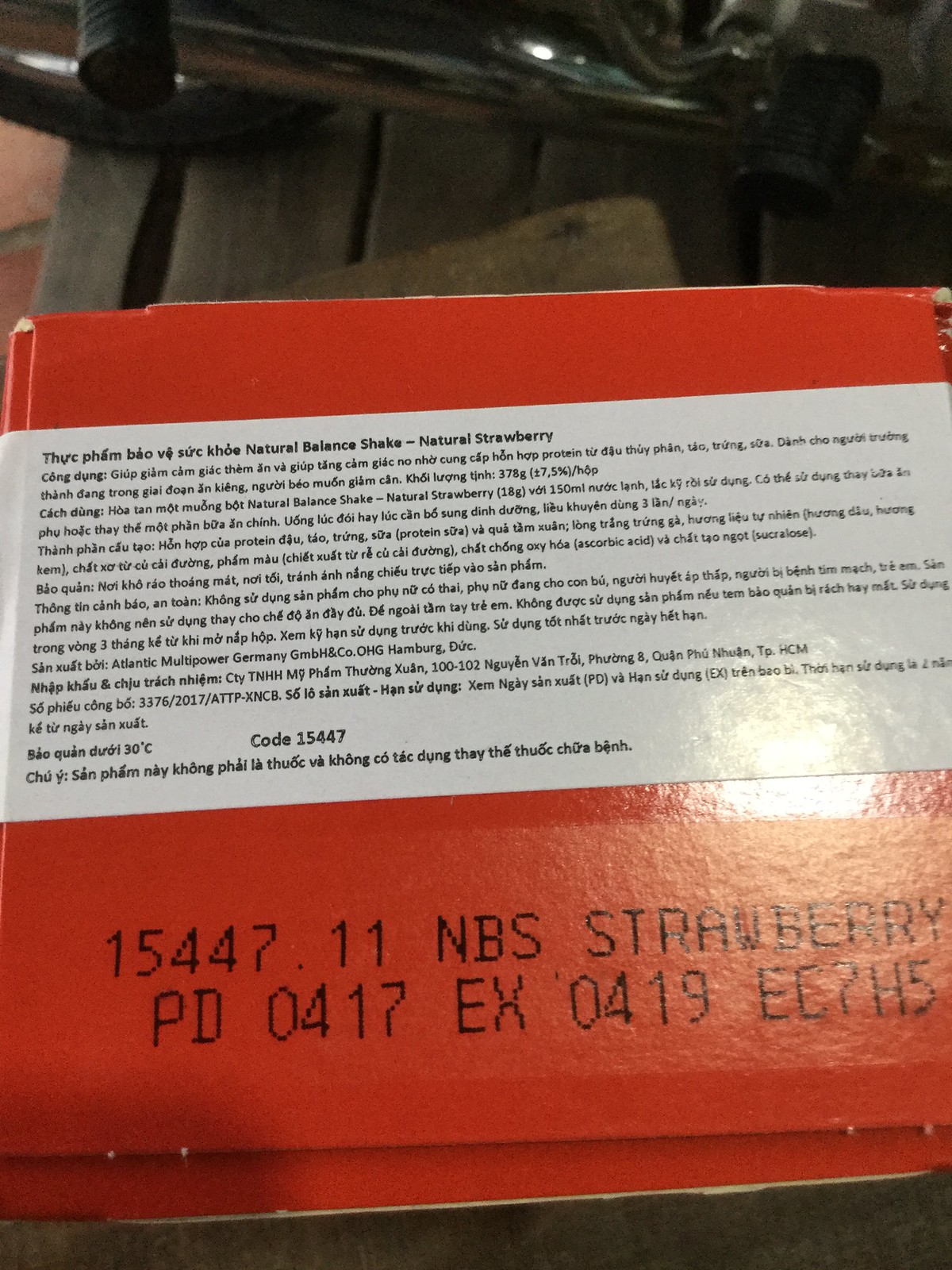The image features the bottom of a white cardboard box presumed to contain an item it was shipped or packaged in. The box itself is predominantly white, adorned with a white label-like tapestry featuring a mix of English and foreign language text. Key details on the label include "Natural Balance Shake" and "Natural Strawberry," indicating the type and flavor of the product inside. Additional text on the box includes the number "15447.11," likely serving as a batch or product code. The initials "NBS" are prominently displayed above a space labeled "Strawberry." Further down, production and expiration date codes are visible as "PD 0417" and "EX 0419." Lastly, a string of characters "?H5" is noted, which could be part of a serial or lot number.